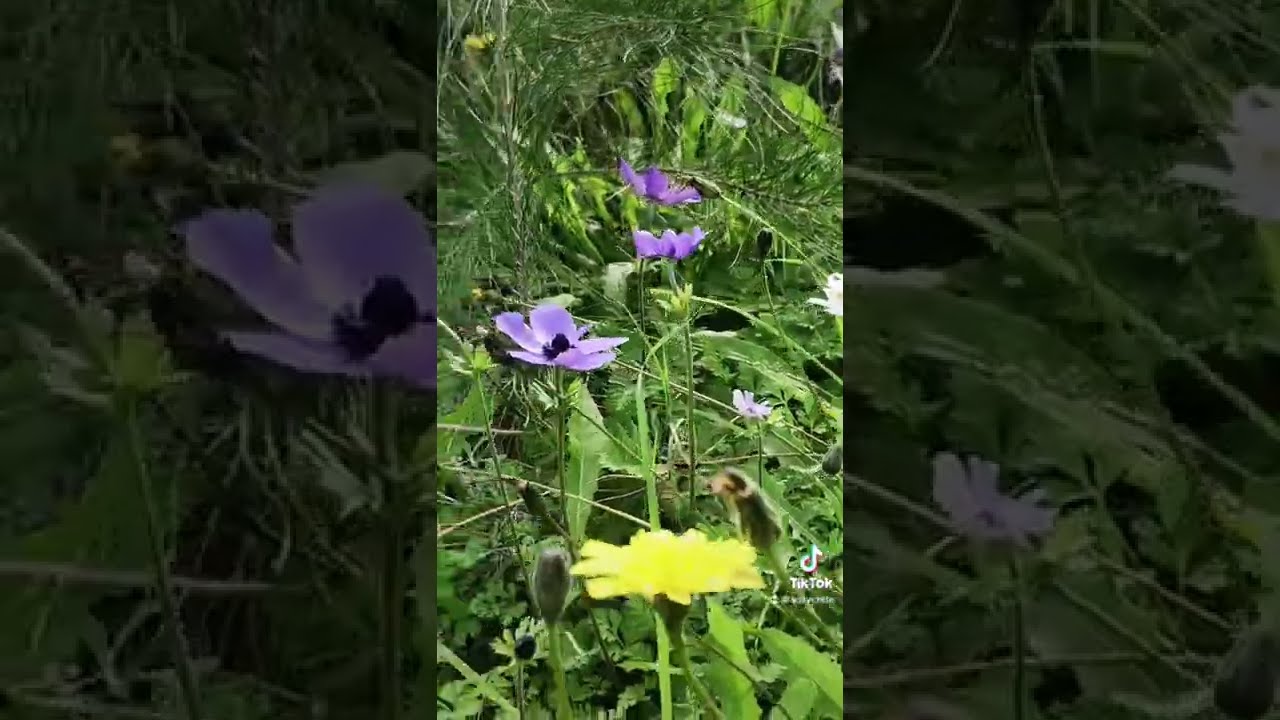The image is a vividly detailed, color photograph captured in portrait orientation, presented as an extreme close-up of various flowers amidst lush greenery. This central photograph is inset into a darkened, landscape-oriented background of the same image. Dominating the foreground at the bottom center is a vibrant yellow flower with a green stem. Just behind it in the middle of the image are three prominent, lavender-colored blooms with black centers, the largest of which is fully open. On the right side of the photograph, there are three flowers with white petals and green stems. Scattered throughout the frame, the background includes additional blooms and branches, lending a realistic and representational feel to the composition. On the right side of the image, in white font, is a music symbol; below that, the text "TikTok" is visible, with additional illegible white text below it.